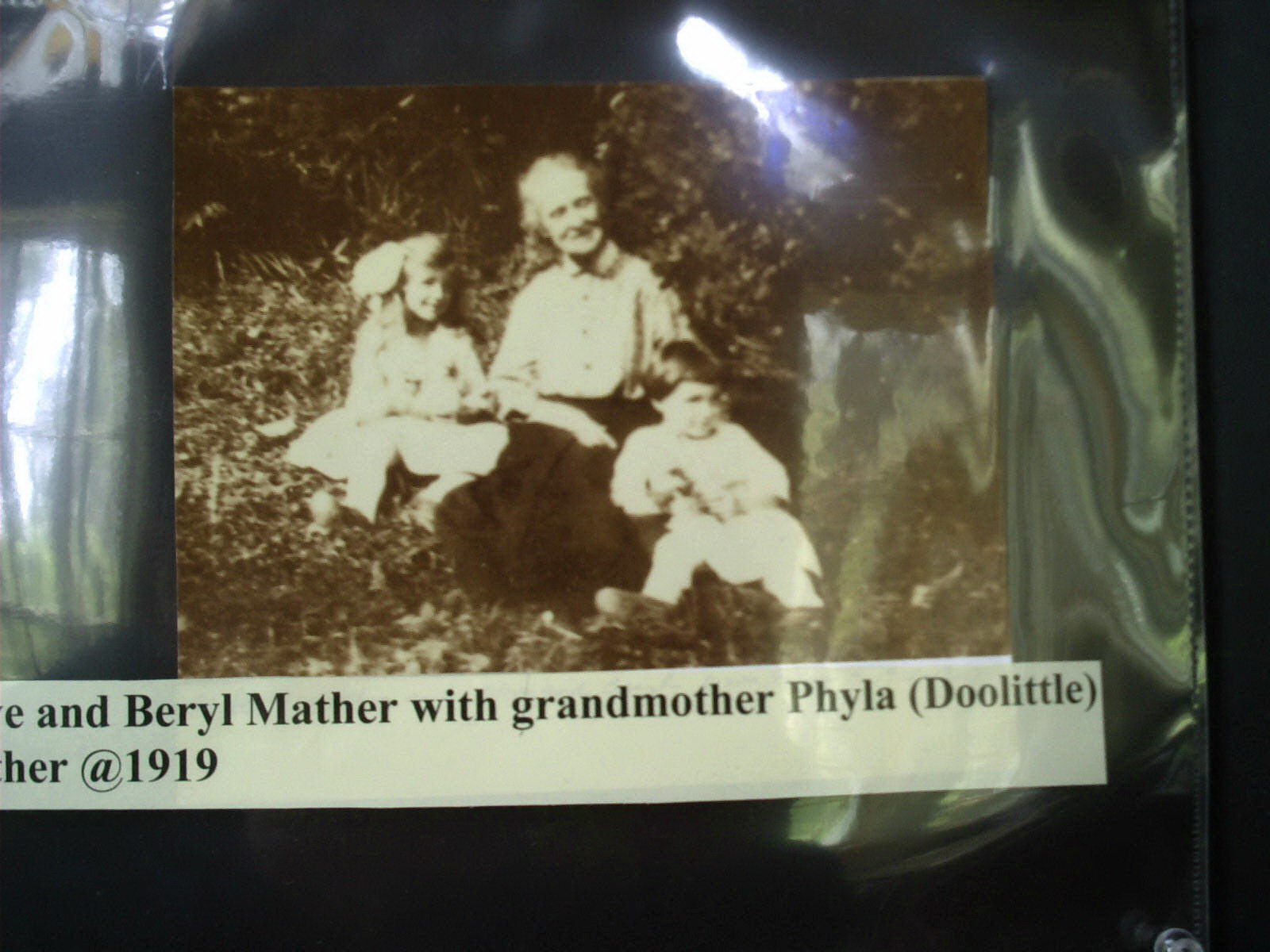This is an old sepia-toned photograph from 1919, encased in protective plastic. It is likely displayed on a bulletin board, partially obscuring a typed note that identifies the subjects. The image captures Grandmother Viola Doolittle who is sitting on the grass among leaves, accompanied by her grandchildren, Beryl Mather and another child.

Grandmother Viola, dressed in a white blouse and a large dark skirt, sits comfortably. To her side is Beryl, a pretty little girl with long blonde hair adorned with a flower. She is wearing a white dress. Beside them is another child, a boy with short dark hair, also in white, holding an unidentified object. The ambiance suggests they are in a park or a wooded area, adding to the rustic and nostalgic feel of this family moment. The overall scene portrays a serene family gathering, frozen in time.